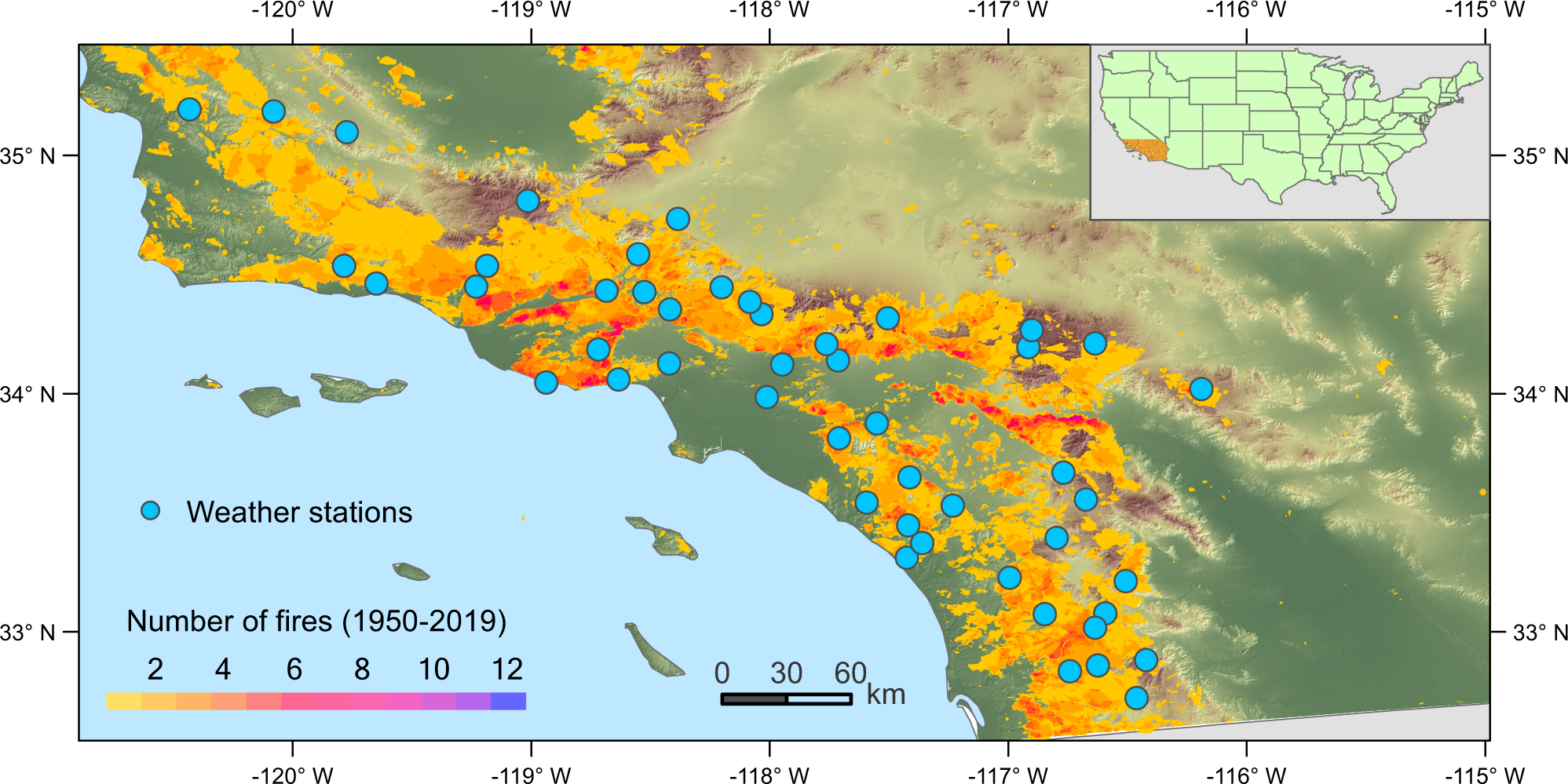The image depicts a detailed map of Southern California, highlighting the region's forest fires and weather stations. The primary map includes a key on the bottom left-hand corner, which uses a chromatic color range from yellow to purple to represent the number of forest fires from 1950 to 2019. Yellow indicates low fire frequency, while purple signifies higher occurrences. Various blue dots across the map denote weather stations. 

A smaller inset map of the entire United States, located in the top right corner, offers a geographic reference for Southern California. The map also features coordinates around its perimeter, with a scale showing distances from 0 to 60 kilometers, and degrees of latitude and longitude marked for precise navigation. The background predominantly showcases green and white areas, with hues of orange, yellow, and purple interspersed to illustrate fire data. The overall composition of the map is rectangular and uses vibrant colors, including various shades of blue for the weather stations.